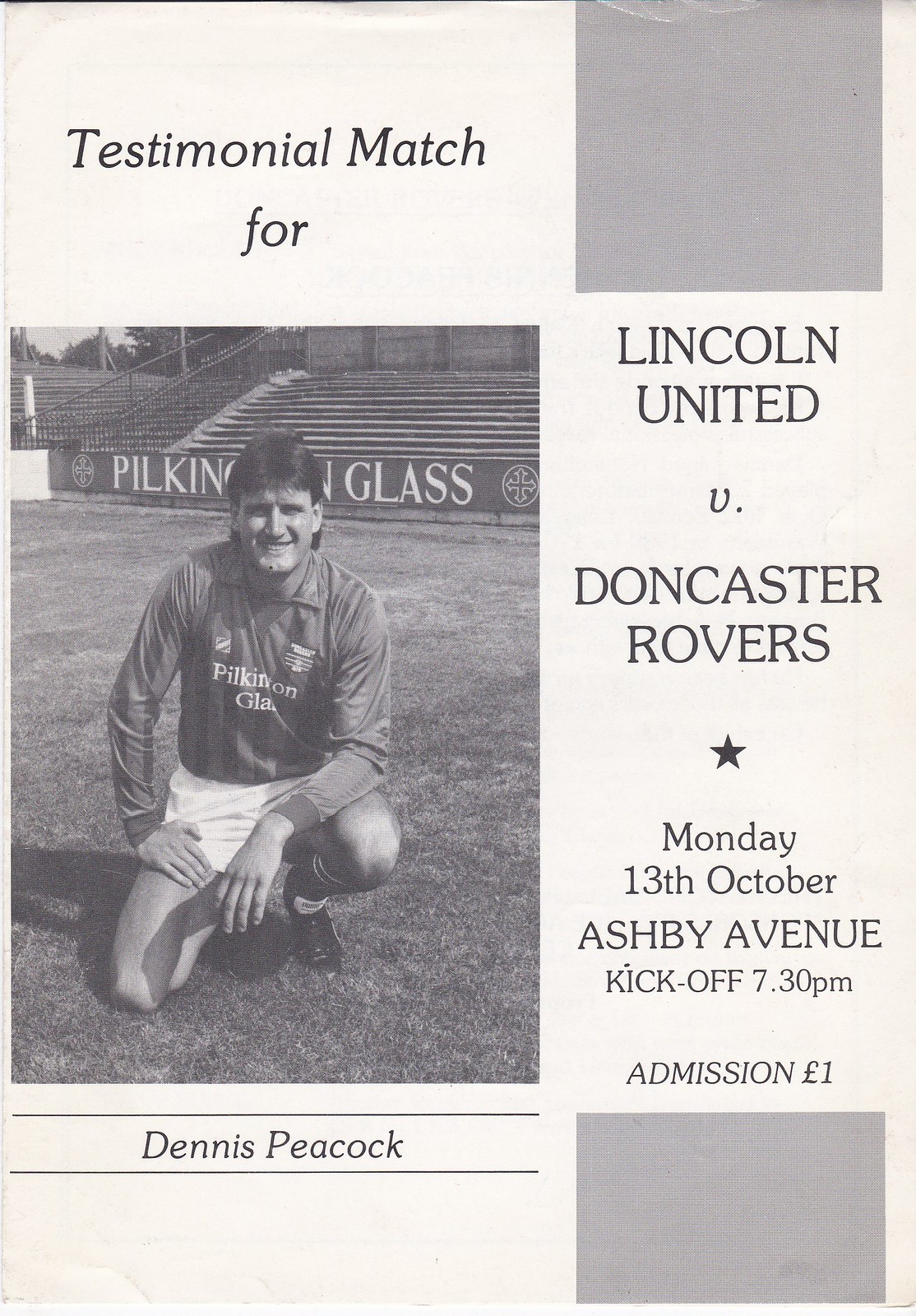The image appears to be the cover of a program for a soccer match. The background is a creamy white color, and the design is entirely in black and white. In the top left-hand corner, it says "Testimonial Match 4" and to its right, "Lincoln United vs Doncaster Rovers." Below these, a black star is featured, followed by details about the event: "Monday, 13th October, Ashby Avenue, kick-off 7.30pm, admission £1." 

On the left side of the cover, there is a black and white photograph of a footballer, identified as Dennis Peacock, kneeling on one knee on the grass. He is smiling and dressed in a long-sleeve, striped football shirt bearing the sponsor's name "Pilkington Glass." Behind him, a banner also displaying "Pilkington Glass" is visible. Underneath his picture, the name "Dennis Peacock" is written in black text. Additionally, there are grey blank squares in the top right-hand and bottom right-hand corners of the cover. This thoughtfully detailed layout emphasizes the significance of the testimonial match for Dennis Peacock.